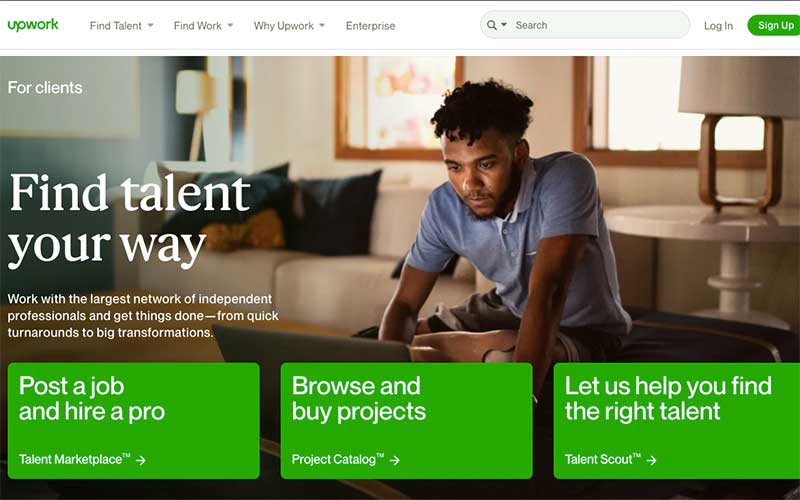This image, sourced from the Upwork website, features a detailed and dynamic homepage layout. In the upper left-hand corner, the "Upwork" logo appears in green. Adjacent to it are drop-down menus labeled "Find Talent," "Find Work," "Why Upwork?," and "Enterprise." Towards the right side of the top navigation bar, there is a search bar, a "Log In" link, and a green "Sign Up" button.

Dominating the central portion of the image is a photograph of an African-American man wearing a blue polo shirt, seemingly engaged in typing on his laptop. The setting suggests a cozy living room, complete with a beige couch adorned with black pillows, a wooden table holding a lamp, and a few visible windows providing natural light.

In the upper right corner, the caption "For Clients" is displayed, while the middle section of the image prominently reads: "Find Talent Your Way. Work with the largest network of independent professionals and get things done—from quick turnarounds to big transformations."

Towards the bottom of the image, there are three green rectangular buttons: the first one reads "Post a Job and Hire a Pro," the second says "Browse and Buy Projects," and the third states "Let Us Help You Find the Right Talent."